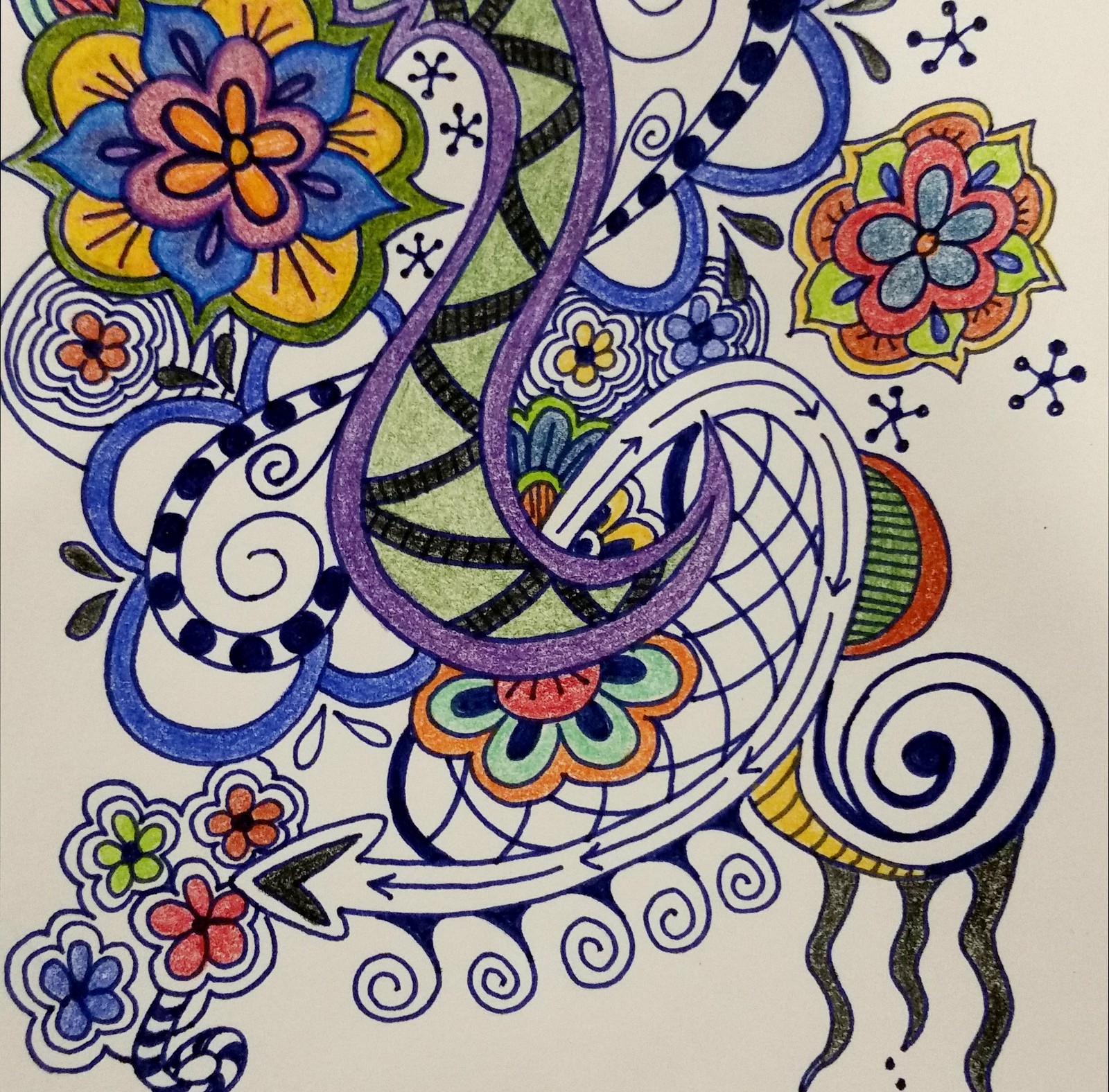This square, intricately detailed, and vibrant doodle appears to have been created on white paper or a sketch pad. Dominating the composition is a wavy, abstract design that curls inward from the center, resembling a snake tail with crosshatched lines. Surrounding this central motif, several vividly colored flowers, each with uniquely shaped petals, float freely, adding to the dynamic nature of the artwork. The design is reminiscent of the late 1960s' hippie aesthetic, featuring a dark blue outline that encapsulates areas filled with a spectrum of colors—likely applied using crayons or colored pencils. A prominent swirl emanates from the main design, ending in an arrow that directs attention from the middle center of the image towards the bottom left, adding an element of direction and movement to the piece.